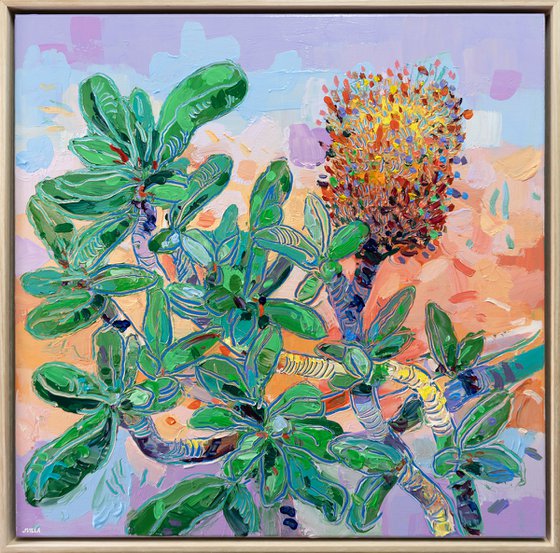This square-shaped painting features a richly textured, jungle-like plant that dominates the canvas. Surrounded by a tan inlaid border and framed in gray, the artwork showcases numerous tubular branches, rendered in varying shades of gray, purple, and brown. Each branch supports clusters of dense, long, oblong, smooth green leaves. Prominently, one branch extends into a vibrant, bushy bloom positioned in the upper right of the image. This bloom resembles a peacock's tail or a powder brush due to its multitude of tiny, colorful flowers in hues of green, red, yellow, purple, blue, and orange. The background of the painting transitions from light purple at the top and bottom to different shades of orange in the middle, providing a striking contrast to the lush greenery. A white artist's signature adorns the bottom of the image, confirming its unique artistic identity.